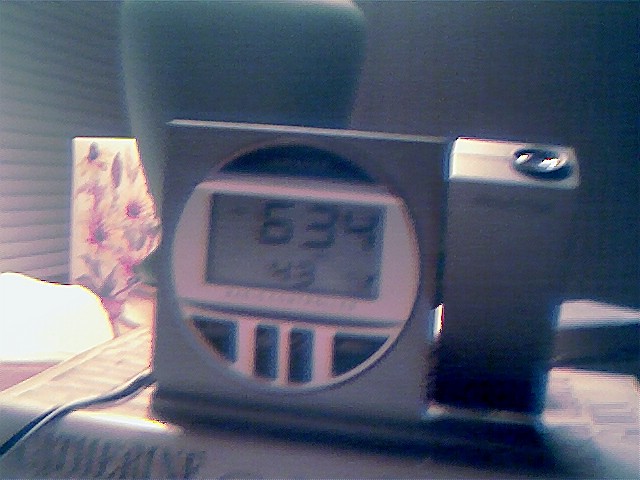The image captures a detailed close-up of an alarm clock resting on a tabletop. Positioned centrally, the alarm clock stands upright, featuring a unique combination of shapes and colors. Its overall form is square, but the clock face itself is circular and outlined in gray, which contrasts with the vibrant blue top. Prominently displayed in the center is a rectangular white digital screen displaying the time "6:34" in bold black text.

Beneath the digital screen are four smaller shapes, each highlighted with blue outer lighting and edges, adding a touch of detail to the clock's design. To the right of the clock face stands a vertically aligned rectangular shape that is blue at the bottom and transitions to gray at the top.

In the foreground, a dark blue and white wire snakes out from the bottom-left corner, likely trailing behind the clock. Behind the clock, a light blue vase provides a subtle splash of color. The majority of the background is muted gray, but there is a hint of blue shading near the top right corner, adding depth to the scene. At the bottom of the image, faint bluish-green letters can be seen, though they appear quite faded. The overall composition is a mix of geometric shapes and soft colors, creating a visually intriguing snapshot of a seemingly mundane everyday object.